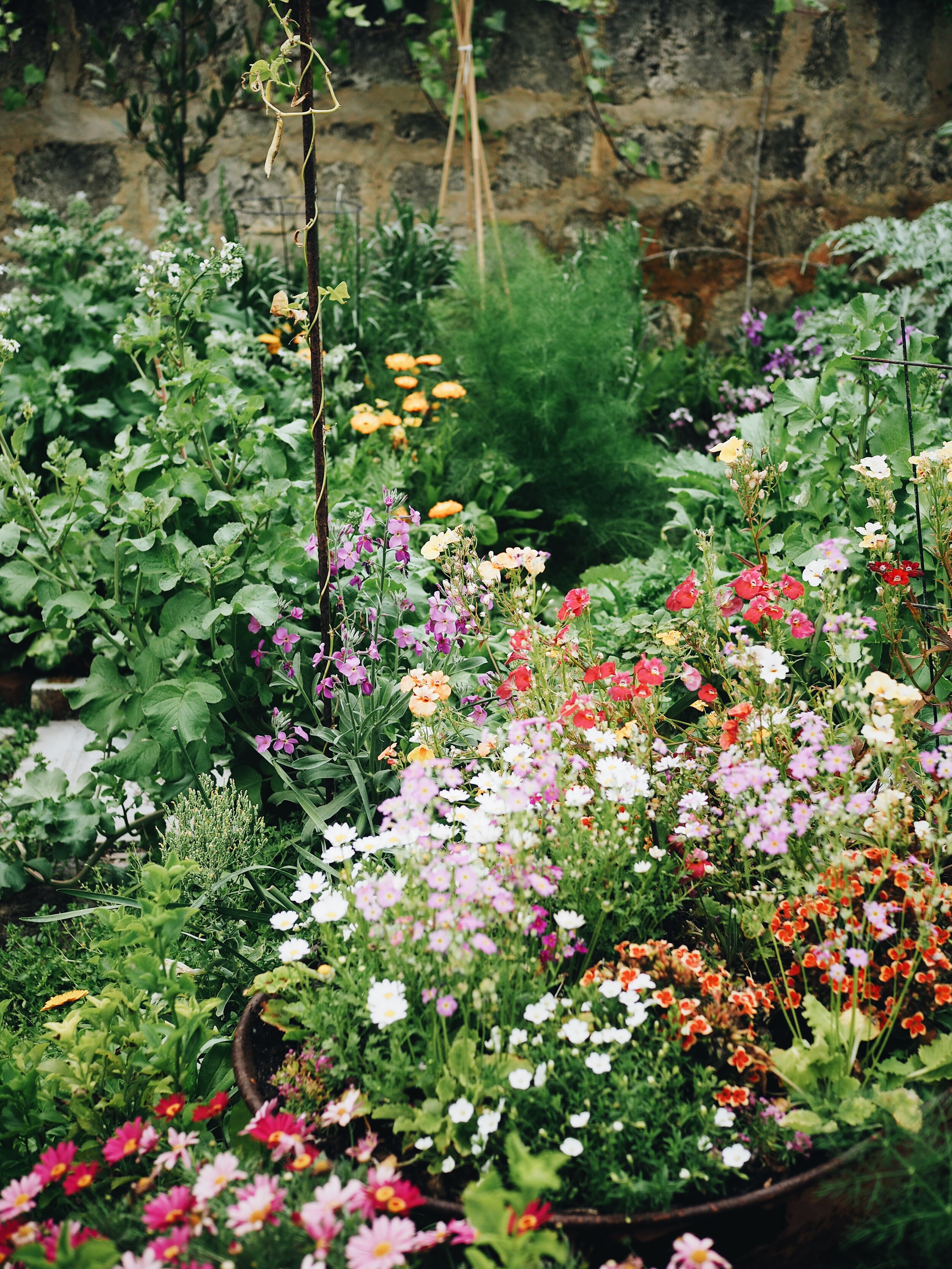This image depicts a vibrant garden scene abundant with various plant life and colorful flowers. At the center, a large, round, flat pot (referred to variously as a pot, dish, and basket) dominates the lower right part of the frame, brimming with an array of small, vividly-colored flowers including red, pink, orange, yellow, white, and purple blooms. These flowers stand out against the predominant lush green foliage that fills the middle and front of the image. Strikingly, a black metal post with beige vines spirals up from the greenery toward the mid-left of the frame. In the background stands an old stone wall, composed of black and gray stones interspersed with stretches of yellowish-beige mortar. Centrally placed against this wall is a pyramidal arrangement of three beige sticks tied together with white string. The detailed textures and colors — from the vividly highlighted flowers to the variegated stones — create a rich tapestry of elements, evoking the quaint, serene beauty of an immaculately tended garden.